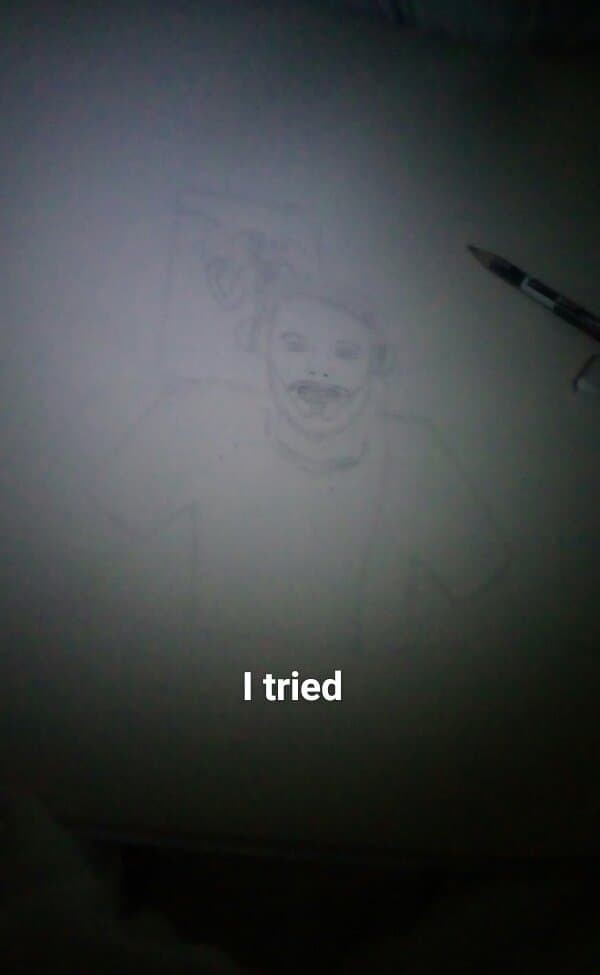This detailed sketch features a middle-aged man with a slightly incredulous expression on his face. His hair is neatly parted from left to right, and he sports a partially drawn beard. The man is wearing a t-shirt, though his arms are not completely visible. The sketch's lines are light, giving it a delicate and unfinished appearance. There is an enigmatic background hint that suggests a picture might be on the wall, but its contents are obscured. The sketched image only partially shows the piece of paper it's drawn on, with darkness encroaching from the bottom. A caption underneath reads "I tried," reflecting perhaps the artist's self-deprecating humor or effort. The whole scene is dimly illuminated, as if by a flashlight with waning battery power, adding an air of mystery to the piece.